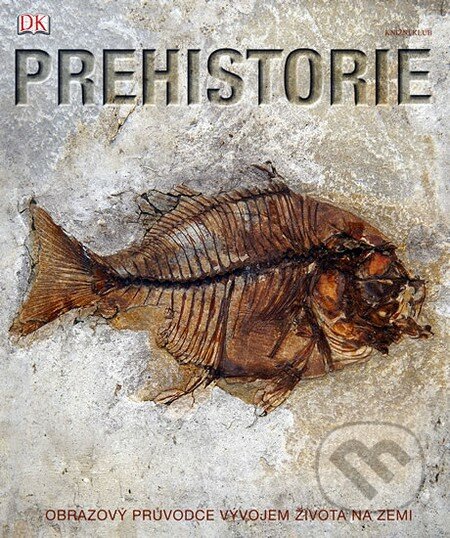This vertically aligned book cover illustration features a textured stone background in swirls of brown and gray, speckled with black. Dominating the center of the cover is a detailed, desiccated fish skeleton oriented to the right, with its fins and tail on the left. The fish, appearing partially mummified or fossilized, is rendered in shades of dark brown and orange, seemingly embedded into the rough stone surface. At the top of the cover, large, bold brown text spells out "Prehistory." In the upper left corner, the red logo "DK" is prominently displayed. At the bottom, dark brown letters read "Obra Zovi, Pruvatsi, Vyvogem, Zivota, Nazemi," providing an intriguing hint of another language.